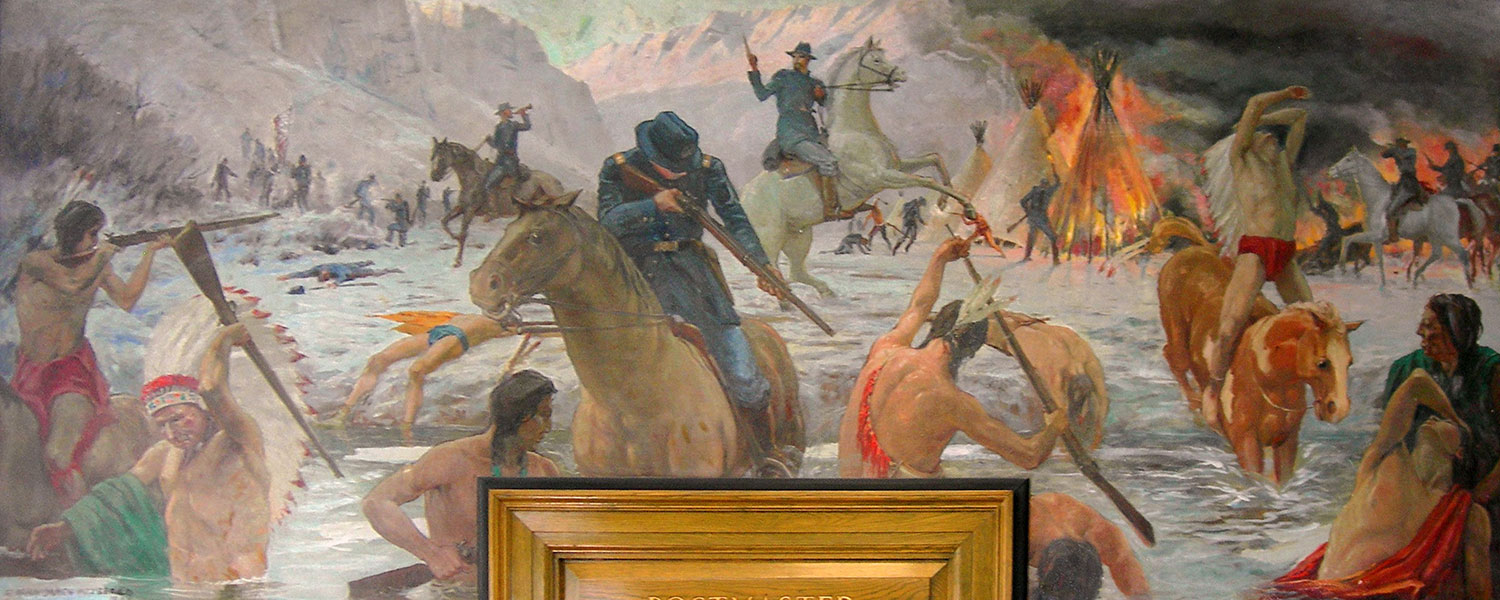The image is a detailed and full-color painting depicting a scene from the American-Indian Wars. It is horizontally rectangular, featuring no definitive border except for a black background over a piece of brown wood shaped like a frame at the bottom center. The chaotic outdoor scene is set against a backdrop of snow-covered mountains. In the upper right-hand corner, billowing black smoke ascends from a tipi engulfed in flames.

The painting vividly captures a fierce battle. United States military personnel, clad in their distinctive blue uniforms, are predominantly mounted on horses, with only a few soldiers visible on foot. In total, there are about six soldiers on horseback. A striking figure in the lower right-hand corner appears to be a Native American chief, distinguished by his elaborate headgear and older appearance. Multiple Native American figures are either on foot or on horseback, with one notably wading in water and holding a gun over his back. The terrain is ambiguous, complicating the differentiation between land and water.

The distressing scene portrays an imbalance, with most Native Americans seen struggling on the ground or in precarious positions, suggesting a dire situation for them. The intensity of the conflict is underscored by the depiction of soldiers actively setting a group of tipis on fire, amid a scattering of small figures in the distant background. The overall atmosphere of the painting is a mix of tension and violence, making it not only visually compelling but also deeply unsettling. The presence of burning structures, men in warfare, and the surrounding harsh landscape captures the grim reality of the historical conflicts represented.